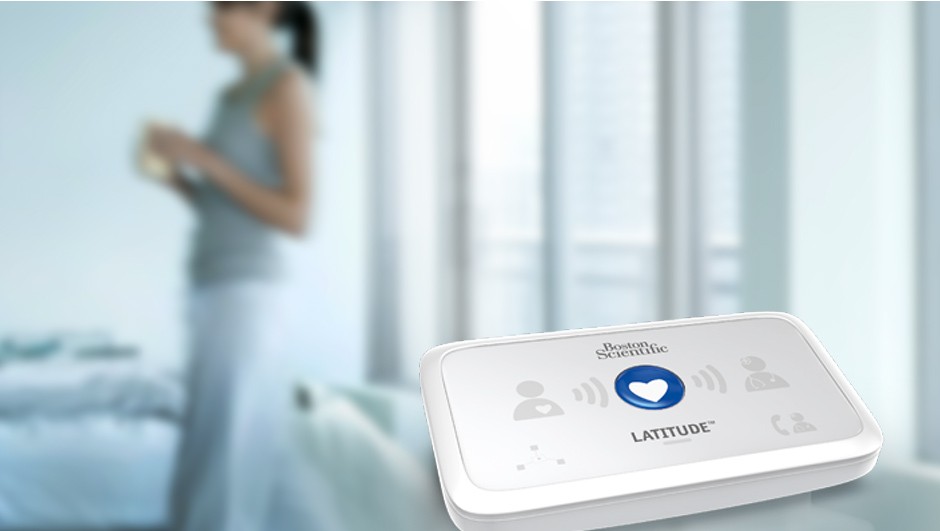The image displays an advertisement set against a soft-focus background of a bedroom featuring long paneled curtains framing a large window. In the mid-ground, a woman with black hair tied into a ponytail, dressed in white pants and a gray tank top, is holding a cup. She appears to be walking away from the window. Dominating the bottom right-hand corner of the image is the product being advertised—a rectangular device labeled "Boston Scientific Latitude." The device features a prominent blue button with a white heart in the center. To the left of the button is an illustration of a patient with a heart symbol, and to the right, a silhouette of a doctor with a stethoscope around his neck. The device, likely an electronic health monitoring instrument, suggests a connection between the patient's heart and the doctor, enhancing remote health management.